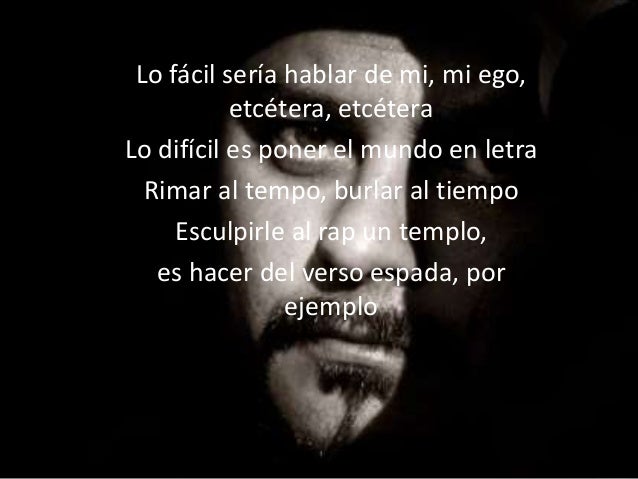In the image, a black-and-white photograph of a man's face is prominently centered against a completely black background. Overlaid on the image, in the center, is text written in a foreign language. The text, appearing in white, spans five to six lines on a medal-like graphic. A rough translation of the text reads: "It is easy, serious, helpful, for me, my ego, etc. It is difficult, yes, the owner, the world, the letter." The positioning and style suggest that the image could be a meme or a motivational message, possibly aimed at social media sharing. The monochromatic color palette of black, white, and shades of gray adds to the somber and reflective mood of the image.